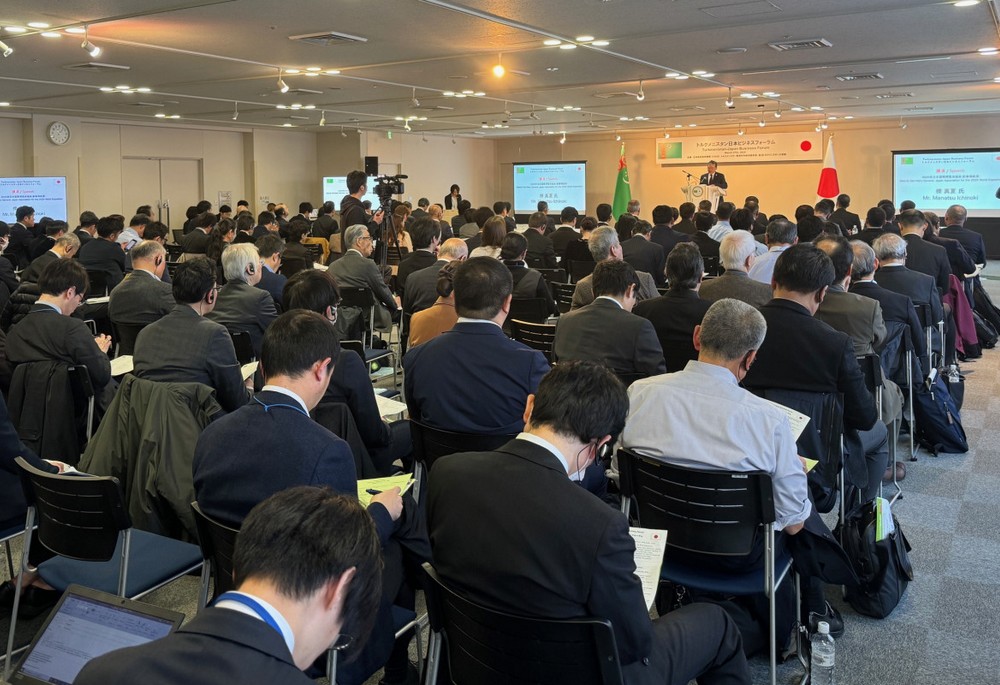In this photograph taken from the back of a conference room, about a hundred attendees, predominantly men in dark suits, are seated in rows of black chairs. Many are looking down at papers or laptops. The room features a checkerboard floor and a ceiling with foam tiles and recessed lighting, indicative of a commercial setting. At the front, a man stands at a podium with a microphone, flanked by two large presentation screens. To his right, a white flag with a red dot, representing Japan, and to his left, a green and orange flag. The overall scene captures a formal atmosphere, with attendees intently focused on the presentation. In the middle of the image, a man with a video camera stands capturing the event.